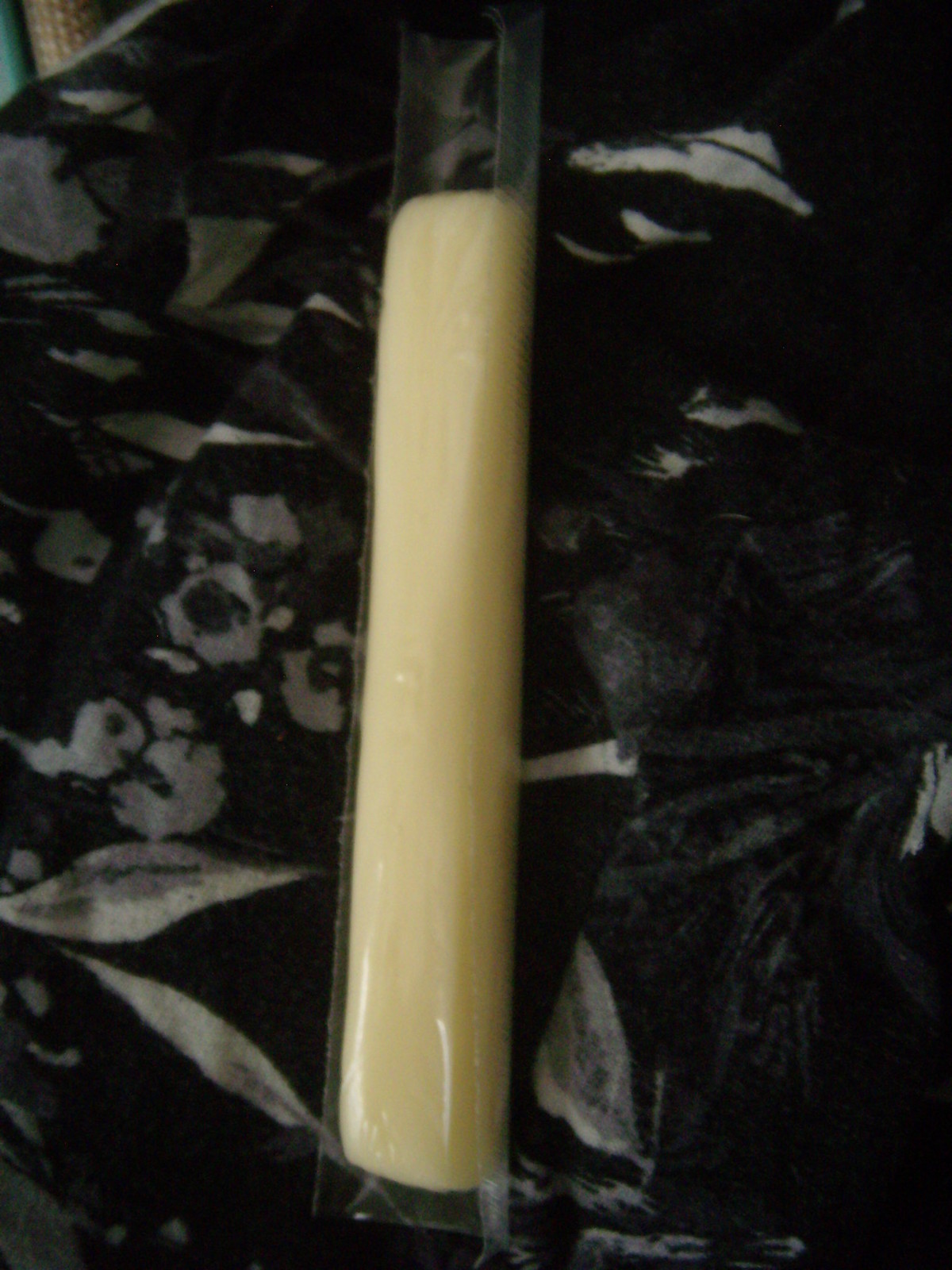The photograph showcases a mozzarella string cheese, still sealed in its clear plastic wrapper, extending from the top to the bottom of the image. The cheese appears intact, with no visible defects or peeling. The background is a dark fabric adorned with intricate white leaf and flower patterns that include round flowers with black centers and oblong leaves. In the upper left-hand corner of the image, there's a hint of something gray, possibly resembling a cup of corn on a turquoise or aqua background. The composition is dominated by the cheese stick, which is prominently displayed against the patterned fabric.